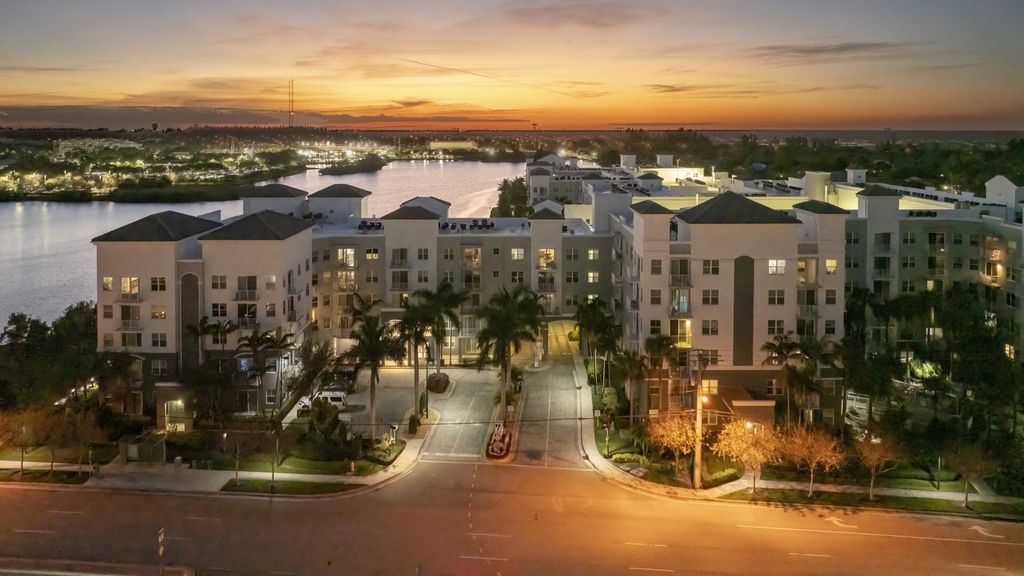This image is an aerial view of a large apartment complex consisting of interconnected buildings, each rising up to five stories tall. The bottom two floors of the buildings are painted gray, while the upper floors are white. The roofs are black and come to a pyramid shape. Well-paved roads covered with gray asphalt lead in and out of the complex, connecting to a larger main road. These roads have clear white markings such as arrows and lines to indicate traffic lanes and directions. Within the image, a parking lot is visible, containing a white SUV and several smaller, dark-colored cars. It's dusk, and most of the apartment lights are on, adding a warm glow to the scene. Surrounding the complex are numerous palm trees along with other smaller trees and lawns, enhancing the overall aesthetic. Additional details of the sunset reveal a beautifully painted sky with hues of orange, red, and yellow, while a river winds its way behind the buildings, offering a picturesque backdrop. The elevated perspective of the image gives a comprehensive view of this well-lit and well-designed residential space, blending seamlessly with the natural and urban landscape.